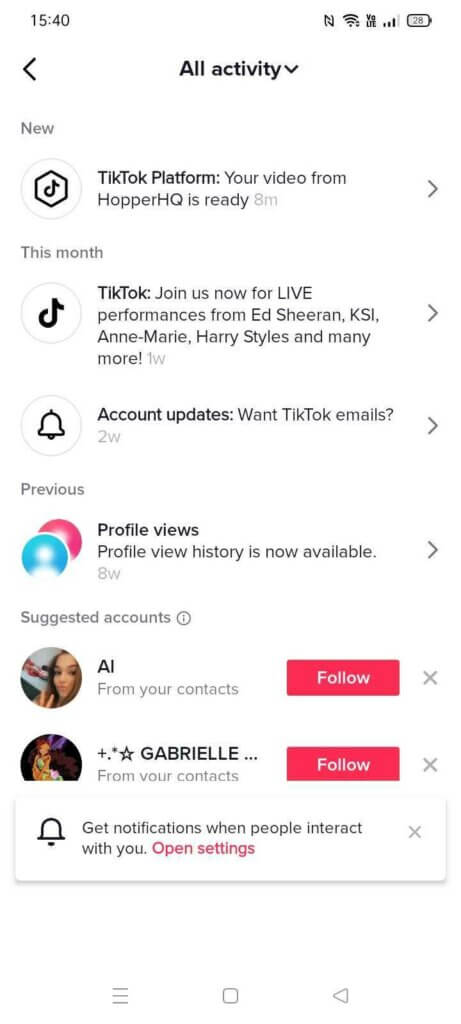This screenshot displays a phone screen featuring TikTok notifications alongside various app icons and status indicators. The time at the top indicates 15:40, with icons signifying internet connection and a battery level at 28%. A left-facing black caret is seen next to the "All Activity" heading, which is accompanied by a down-facing caret. 

The notification list begins with the headline "New," accompanied by a hexagon encircling the TikTok logo. It reads, “TikTok platform: Your video from Hopper HQ is ready—8m,” followed by a right-facing caret. 

Next, under the headline "This Month," a notification within a circle featuring the TikTok logo announces, “TikTok: Join us now live for live performances from Ed Sheeran, KSI, Anne-Marie, Harry Styles, and many more—1w,” also followed by a right-facing caret.

Another notification, under the "Account Updates" heading, features a bell icon encircled and reads, “What TikTok emails?—2w,” complete with a right-facing caret.

"Previous" headlines the next section, showcasing a pink circle behind a blue silhouette of a person, stating, “Profile Views: Profile view history is now available—8w,” with a right-facing caret following.

Under "Suggested Accounts," a small eye icon is present. A notification displays a young lady making a peace sign; she appears to be a racially ambiguous young woman, labeled as "AI from your contacts" with a pink "Follow" bar and an X beside it. Beneath, an animated fairy icon next to the name "Gabriel" (highlighted in capitals) also shows "From your contacts," along with a pink "Follow" bar and an X to its right.

The view cuts off the remaining notifications, but at the bottom of the screen, there's a bar stating, "Get notifications when people interact with you," with a pink "Open Settings" button and an X to dismiss.

Overall, this detailed screenshot captures a focused perspective on the TikTok app's notification interface amid other phone status details.